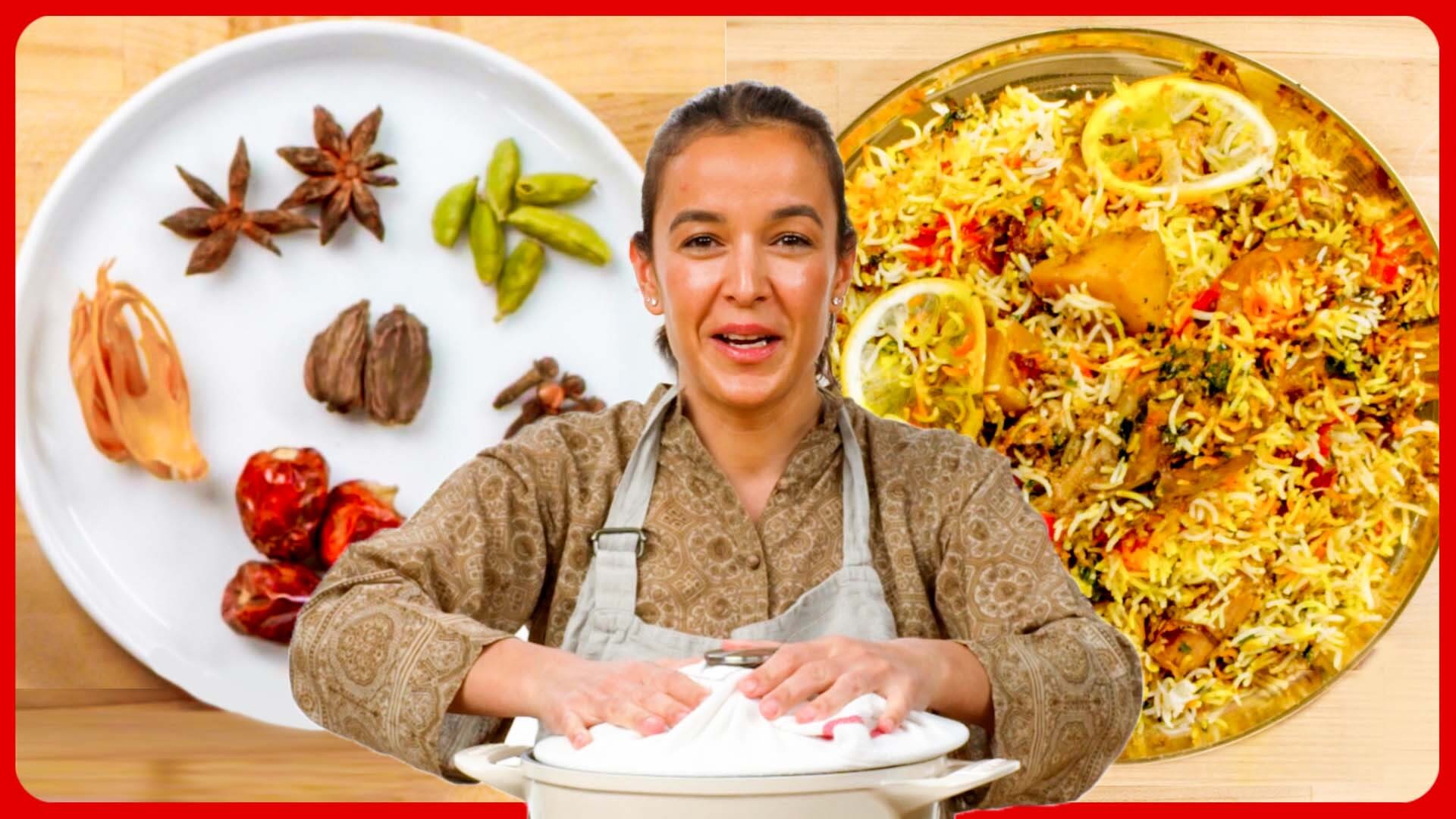In this close-up photo, a smiling white woman with dark hair pulled back in a bun stands at the center, seemingly caught in mid-conversation. She's wearing a brown long-sleeve shirt and jean overalls. She is holding a white Dutch oven pot. Behind her, there is a wooden table with two plates. The plate on the left displays an assortment of spices, including star anise, cloves, green and red chili peppers, cardamom, and other unidentified herbs. The plate on the right features a vibrant yellow basmati rice dish mixed with chunks of chicken, garnished with slices of onions or lemons and drizzled with chili sauce.